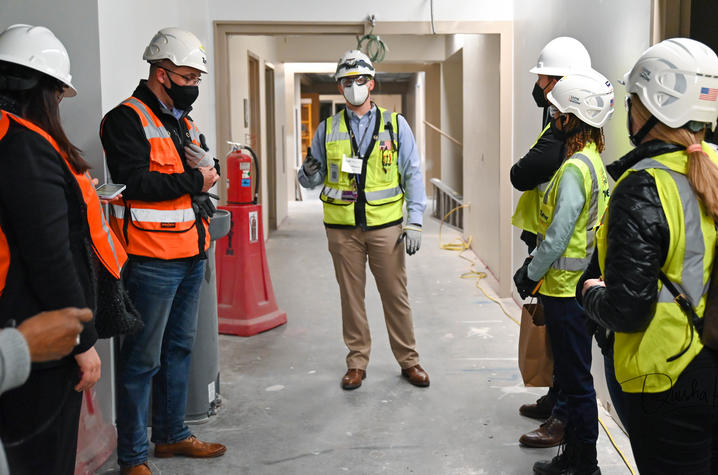In this image, we observe a safety inspection or meeting taking place in a long, seemingly unfinished hallway of a building under construction. The scene is filled with various details: a group of workers all donning white helmets adorned with the United States flag, high-visibility vests, and masks of various colors. The vests are either neon yellow or orange, with most workers wearing blue jeans or khakis paired with long-sleeve shirts. The central figure, who appears to be the supervisor or leader, stands alone in the middle of the hallway, directly facing the camera. This individual wears a yellow vest, a blue shirt, blue gloves, tan pants, and brown dress shoes. Surrounding the leader, the workers are split into groups on either side—three people on the right and two on the left. The right group includes two women and a man, while the left group has a woman and a man. The hallway itself shows signs of ongoing construction: visible construction dust on the ground, wires hanging from the ceiling, and an orange fiberglass ladder in the distance. Additionally, a red fire extinguisher is mounted on a red plastic plinth near the central figure, highlighting safety preparedness. An extension cord can also be seen plugged into the wall and trailing towards the foreground, further emphasizing the work-in-progress nature of the building. This detailed snapshot captures the intense focus on safety and coordination among the construction crew.